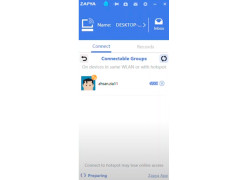This image features a screenshot of a small mobile application interface with the title "Zappa" displayed in white text at the top left. To the right of the title, a sky-blue emblem is visible, followed by a flag-like icon. Several other symbols are arranged adjacent to these, culminating in a white 'X' button situated at the top right corner.

Moving downwards, the left side beneath the title bar showcases an image of a white desktop PC. Adjacent to this image is additional text, and further to the right of this text, there's an inbox symbol accompanied by the word "Inbox" in white text.

Below this section, the interface presents a navigation bar with tabs, including a "Contacts" tab and another indistinguishable tab due to the image's blurriness. 

On the lower section of the interface, there are more elements in blue text. An icon representing a person is located around the center-left area. The remainder of the bottom half of the image is filled with a blank, grayish-white background.